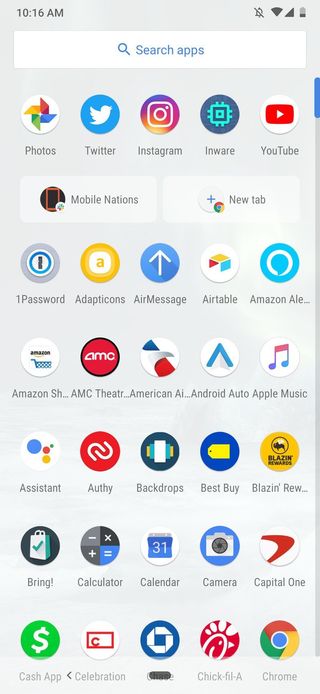The image shows a smartphone screen displaying the home page at 10:16 AM. The status bar at the top indicates no notifications are present, decent internet coverage, and a low battery life, estimated to be 25% or less. The background of the phone is gray, complementing an array of app icons neatly organized in rows. At the top of the screen sits a white search bar for app exploration.

The first row of apps includes:
- **Google**: Represented by the familiar 'G' logo.
- **Google Photos**: Icon depicting a colorful pinwheel.
- **Twitter**: Featuring the iconic blue bird.
- **Instagram**: Displaying the vibrant, gradient camera.
- **InWare**: Marked by technical imagery.
- **YouTube**: With its classic red play button.

Below, in a sort of rectangle format, there are:
- **Mobile Nations**: Iconography unknown.
- **New Tab**: Iconography unknown.

Following are more app icons:
- **Password**: Associated with security or password management.
- **Adaptations**: Specific details unclear.
- **Air Message**: Icon showing messaging features.
- **Airtable**: Noted for project management and databases.
- **Amazon L**: Partially shown, presumably Amazon Alexa or similar service.
- **Amazon SH**: Likely Amazon Shopping.
- **AMC Theaters**: Cinema-related app icon.

Another row features:
- **American Airlines**: Blue eagle logo.
- **Android Auto**: Car symbol indicating in-car connectivity.
- **Apple Music**: Notable music note icon.

Continuing with the next row:
- **Assistant**: Google Assistant with its vibrant dots.
- **Authy**: Two-factor authentication marked by a key.
- **Backdrops**: App for wallpapers and aesthetics.
- **Best Buy**: Blue price tag icon.
- **Blazin Brew** and **Blazin Rewards**: Both associated with a flame, likely tied to a food or drink reward system.

Further down the screen:
- **Bring**: Grocery shopping list icon.
- **Calculator**: Standard calculator image.
- **Calendar**: Traditional calendar grid.
- **Camera**: Depiction of a camera lens.
- **Capital One**: Banking app with an upward swoosh logo.

Finally, on the bottom row, are:
- **Cash App**: Dollar sign in a square.
- **Celebration**: Specific details unclear.
- **Chick-fil-A**: Red and white chicken logo.
- **Chrome**: Renowned colorful round browser icon.

Overall, the screen is densely populated with a wide variety of applications reflecting diverse user needs from social media and productivity to shopping and entertainment.